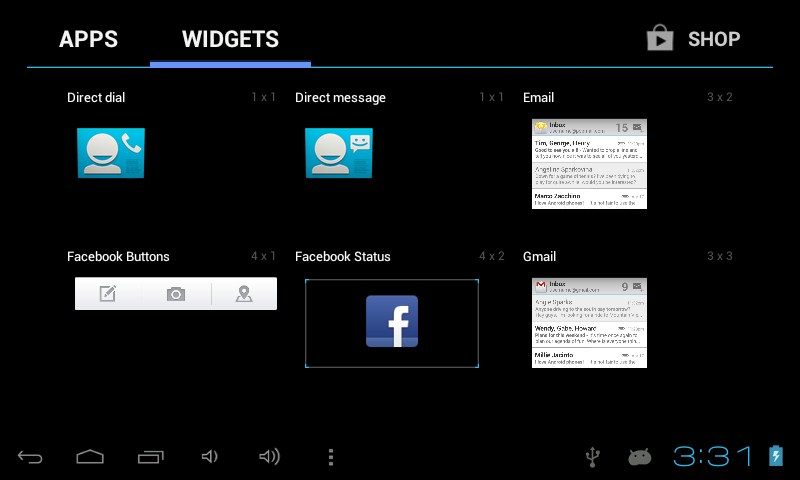The image appears to be a screenshot of a mobile device interface, possibly from a phone or tablet. At the top, there are two tabs labeled "Apps" and "Widgets," with the "Widgets" tab currently selected. In the top right corner, there is an option to go to the "Shop," accompanied by a shop icon. The middle section of the image showcases six widget options: "Direct Dial" with a person and phone icon, "Direct Message" with a person and text icon, "Email" with an email inbox icon, "Facebook Buttons" with multiple icons, "Facebook Status" with the Facebook logo, and "Gmail" with a Gmail inbox icon. At the bottom part of the interface, the main menu features various icons, including the Android icon, USB icon, battery charging icon, and the current time displayed as 3:31 in blue text. Additionally, there are navigation icons like the back icon, home icon, recently opened apps icon, volume controls, and a menu icon represented by three dots.